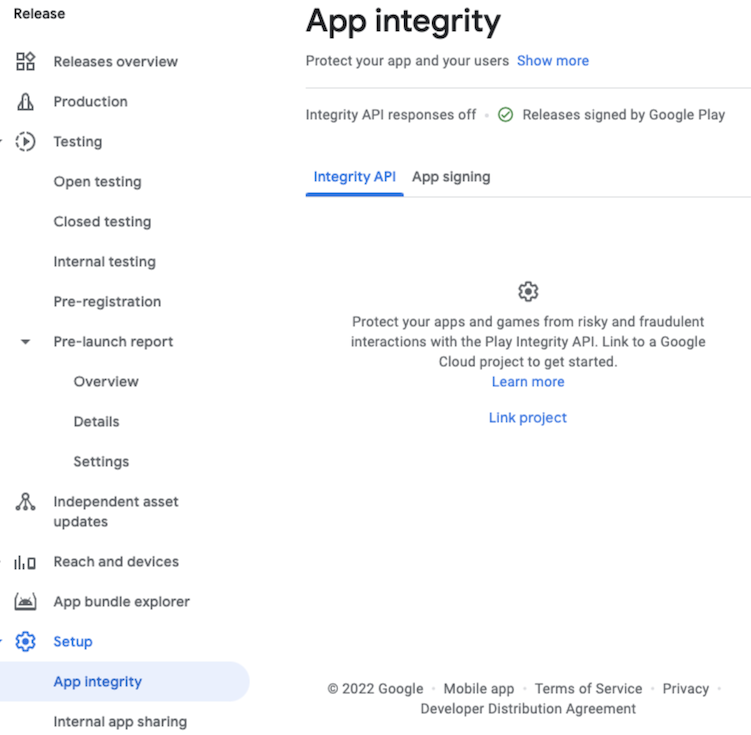This image showcases a screenshot set against a solid white background. In the upper left corner, there is a navigation area featuring the word "Release" in bold, dark gray text. Below this heading, there is a vertical menu listing various sections in descending order: "Releases Overview," "Production," "Testing," "Open Testing," "Closed Testing," "Internal Testing," and "Pre-registration." Further down, the menu includes "Pre-launch Report," which expands into options like "Overview," "Details," and "Settings." Following that, there are additional sections labeled "Independent Asset Updates," "Reach and Devices," and "App Bundle Explorer."

Highlighted in a light blue box is "Set up App Integrity," presented in blue text with a corresponding blue icon. Below this highlighted option, the menu concludes with "Internal App Sharing."

To the right and centered at the top, bold black text reads "App Integrity." Directly below this, in smaller gray text, is the phrase "Protect your app and your users." There is also a blue link to the right saying "Show more." At the bottom of the screenshot, it is indicated that the information is from "2022 Google."